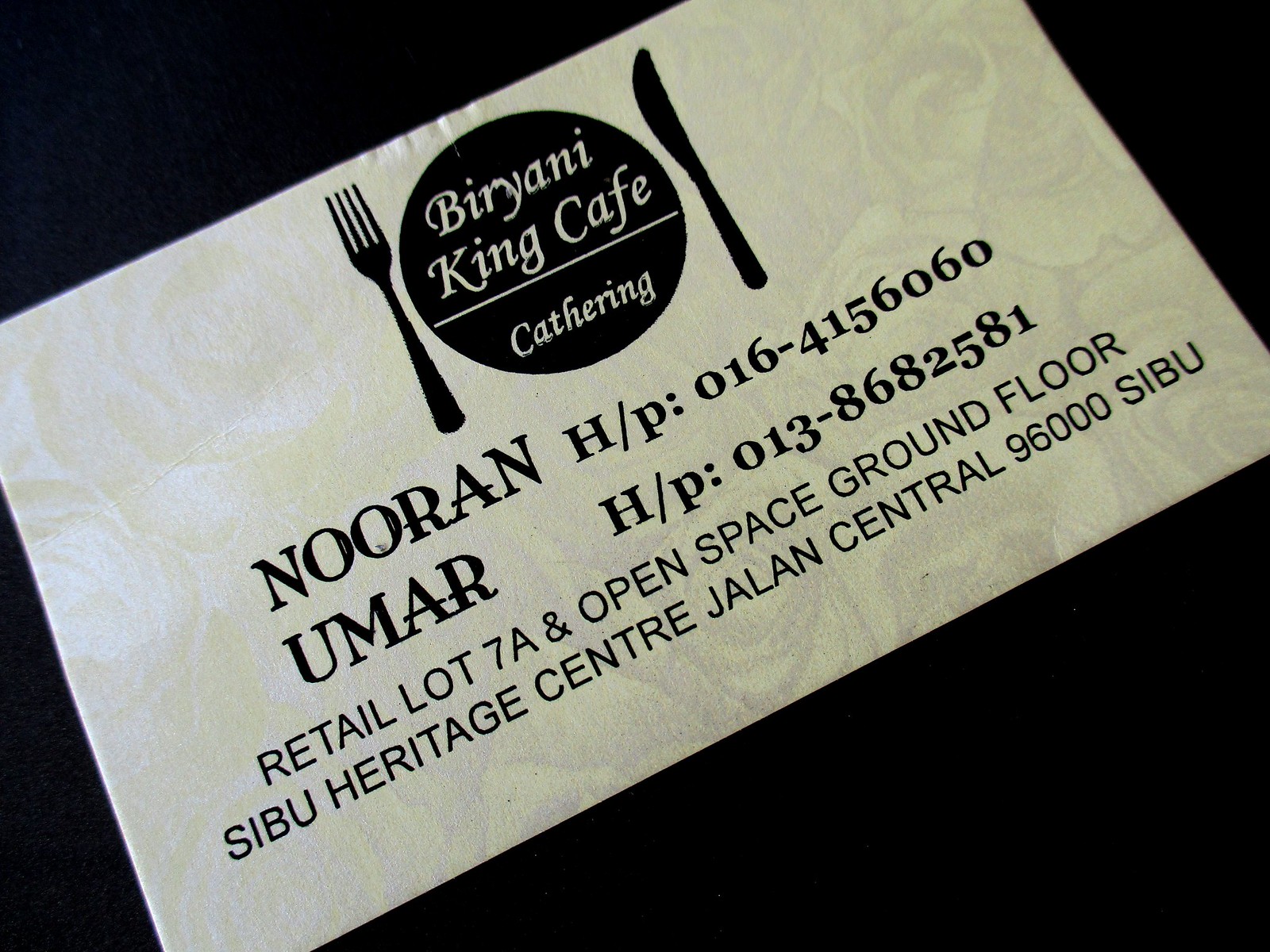This image depicts a white business card with a clear modern design, resting on a black background. The card features a subtle floral pattern in the background. Centered at the top is a black illustration of a fork, plate, and knife. Inside the plate, in clean white text, it reads "Biryani King Cafe" with "Catering" beneath it. Below this central design, the card lists the contact details in black text, starting with the name "Nuran Umar" followed by "H/P: 016-415-6060". Another phone number is listed beneath: "H/P: 013-8682581". At the very bottom, the card provides the address, stating "Retail Lot 7A, Open Space Ground Floor, Cebu Heritage Center, Jalan Central, 96000 SIBU".